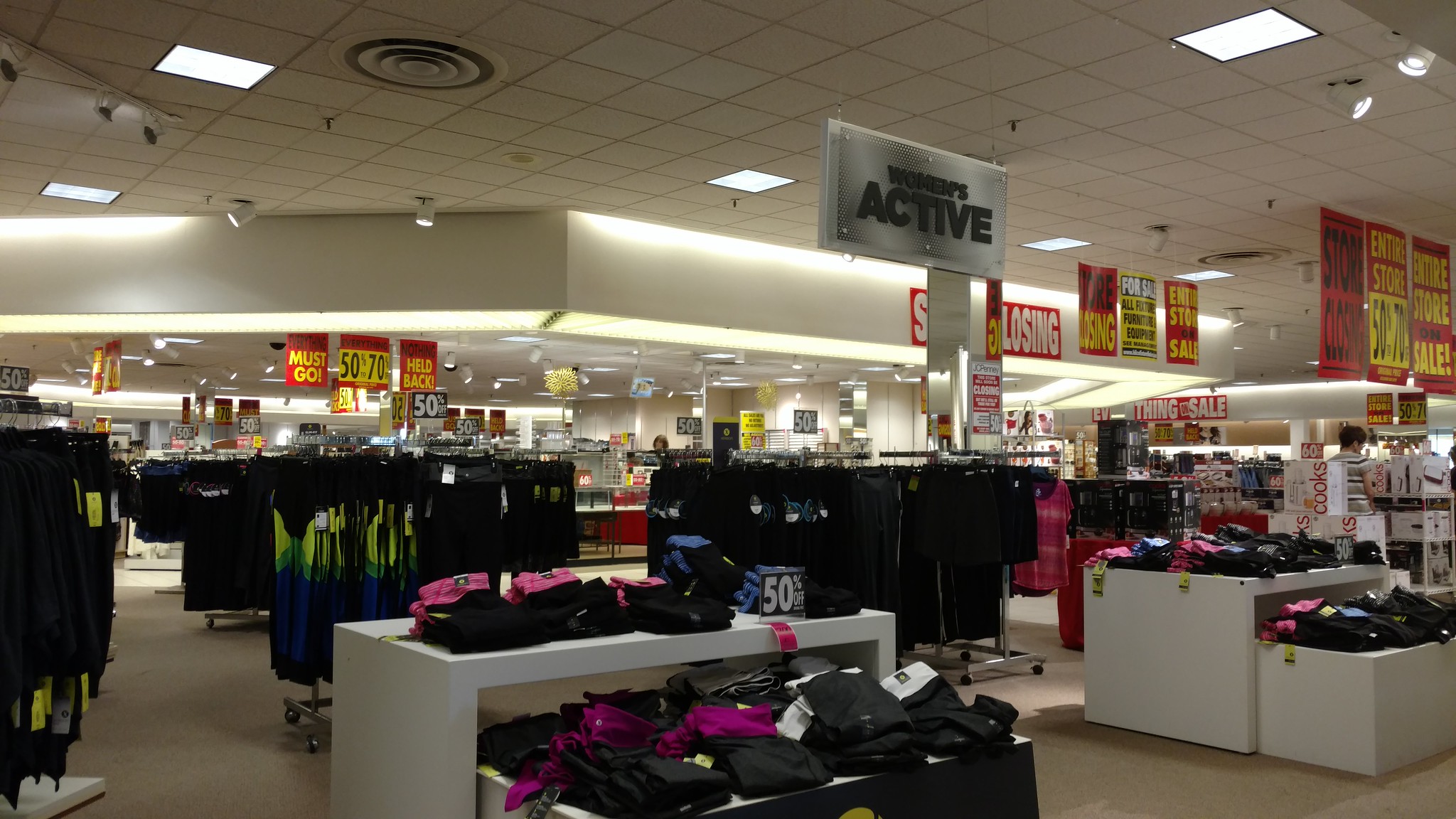The image depicts a spacious retail store interior, brimming with various clothing displays. The tiled ceiling is punctuated by numerous lights, providing ample illumination. Multiple sections of the store prominently feature black clothing items on display. In the foreground, there are white shelves stacked neatly with folded clothes; one shelf is centered in the image, while another is positioned to the left.

Hanging from the ceiling, several signs are visible. A prominent white sign in the center reads "Women's Active" in black lettering. Scattered throughout the store, bright red signs with bold yellow fonts announce a significant sale: "Store Closing," "Entire Store 50-70% Off," and "Everything Must Go, Nothing Held Back." These signs are ubiquitous, emphasizing the store's final clearance sales.